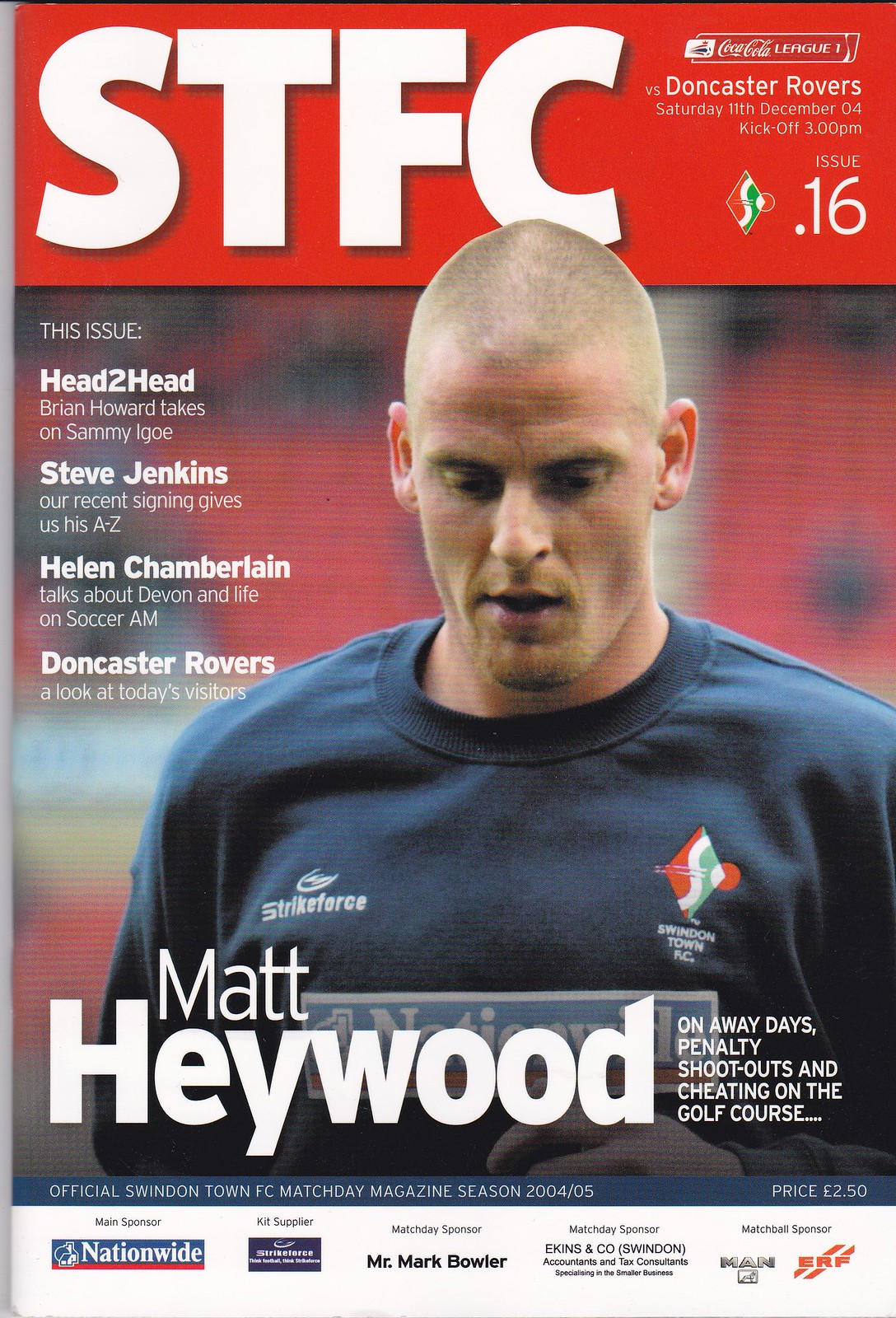The cover of a soccer magazine, issued on Saturday, December 11, 2004, highlights several features and key figures. At the top, within a red border, it states "STFC versus Doncaster Rovers," for a 3 PM kickoff in the Coca-Cola League One, identified by the Coca-Cola logo in the top right corner. This is issue 16. Matt Haywood, depicted on the cover wearing a blue long-sleeve shirt emblazoned with "Strike Force" on the right side of his chest, is featured prominently against a blurred stadium background. The magazine teases various articles inside, including a head-to-head between Brian Howard and Sammy Eagle, an A-to-Z with the newly signed Steve Jenkins, Helen Chamberlain discussing Devon and life on Soccer AM, and an insightful look at the visiting Doncaster Rovers. Additional content includes Matt Haywood on away days, penalty shootouts, and cheating on the golf course. The cover also displays sponsors such as Nationwide, Mr. Mark Bowler, and the price of £2.50. The text is primarily in white.